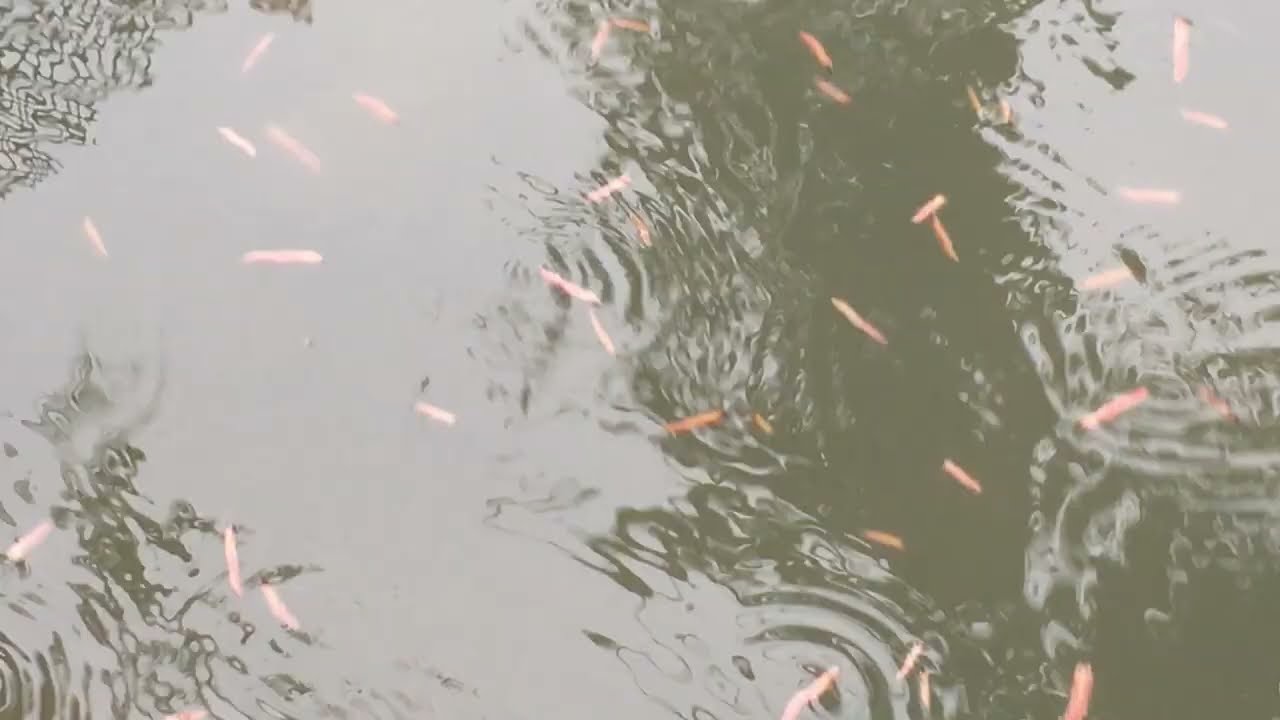The image appears to be a highly zoomed-in and abstract depiction of water with a murky gray and olive greenish hue, reminiscent of army green. The water's surface is characterized by a mix of rippled and unrippled areas, adding an element of mystery. Scattered across the scene are numerous small, pinkish spots that resemble tiny fish or floating debris, numbering around thirty. Some ripples form circular patterns, akin to those created by water droplets, while other areas exhibit jagged, graph-like lines, further complicating the image's interpretation. The overall effect is ambiguous, making it hard to distinguish if this is a satellite image of a planet, an abstract painting, or a unique photograph capturing reflections or distortions on the water's surface.